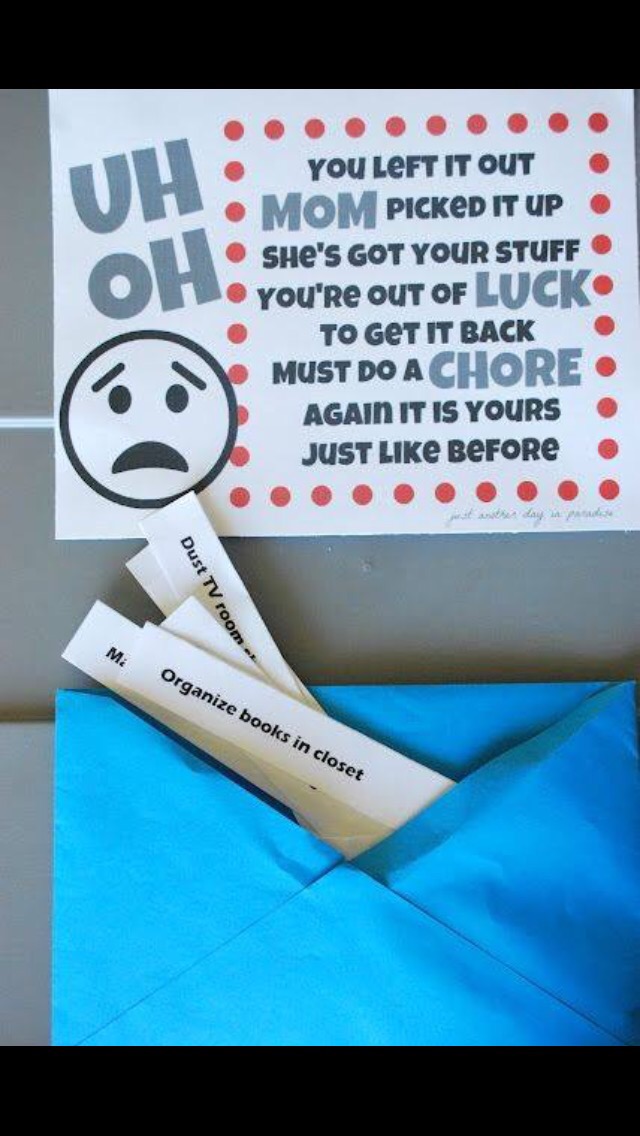This advertisement features a poetic, humorous reminder to children about the consequences of not tidying up. The rectangular, vertically oriented design is bordered by black bars at the top and bottom, with a gray background in between. Central to the image is a white statement area, creatively displaying the text in black and gray. 

At the top of the statement, stylized lettering spells out "uh-oh," accompanied by a distressed emoticon-like face composed of black ovals for eyes, inverted quarter circle eyebrows, and a red-bordered rectangular mouth. Below this, the admonishing text reads: "You left it out. Mom picked it up. She's got your stuff. You're out of luck. To get it back, you must do a chore. Again, it is yours just like before."

Beneath this white sign is a blue envelope, out of which protrude multiple white task slips, appearing like tickets. The first visible slip reads "Organize books in closet," followed by others like "Dust TV room." These slips represent various chores, neatly stacked and pointing upwards at an angle, reinforcing the playful yet instructive message of the advertisement.